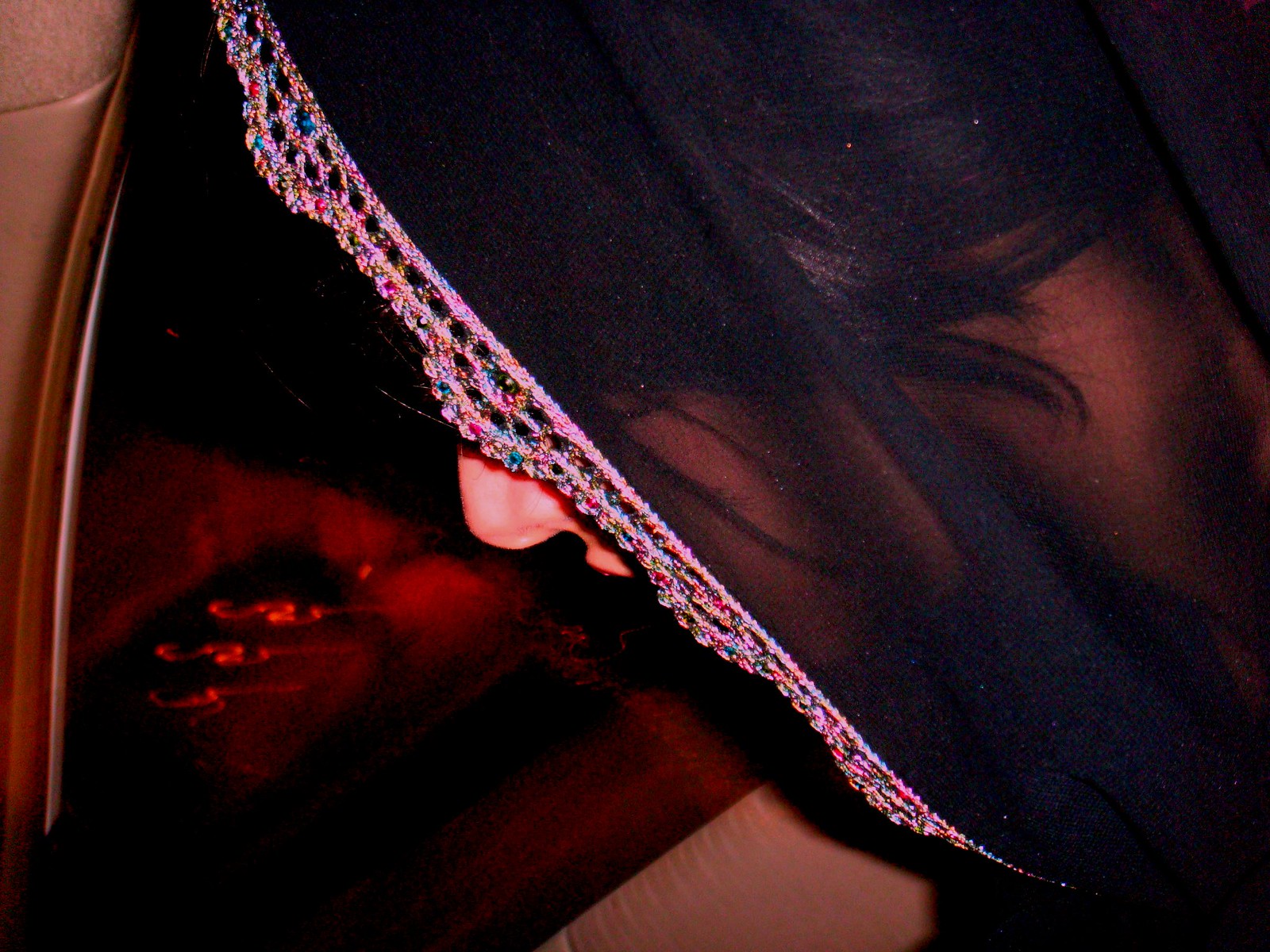This image appears to be a close-up of the left side of a woman's head, slightly dark and a bit blurry. She is adorned with a black lace veil featuring a decorated trim that seems to include jewels and possibly some pink and multicolored elements. Her black hair can be seen beneath the veil, along with part of her profile and the back of her neck. The woman is leaning over, closely examining some objects in front of her, potentially within an indoor setting that includes minimal lighting. 

In the foreground, there appears to be a brown wooden base containing three S-shaped items that resemble necklaces with pendants. Just below this wooden structure, some white fabric is visible. Adding to the scene's complexity, there is a suggestion of a fireplace or brick oven to the left, emitting bright orange embers. Although it is unclear exactly what she is doing, the woman is looking downward, focused intently on something other than the fireplace, perhaps indicating a moment of quiet contemplation or intricate work.